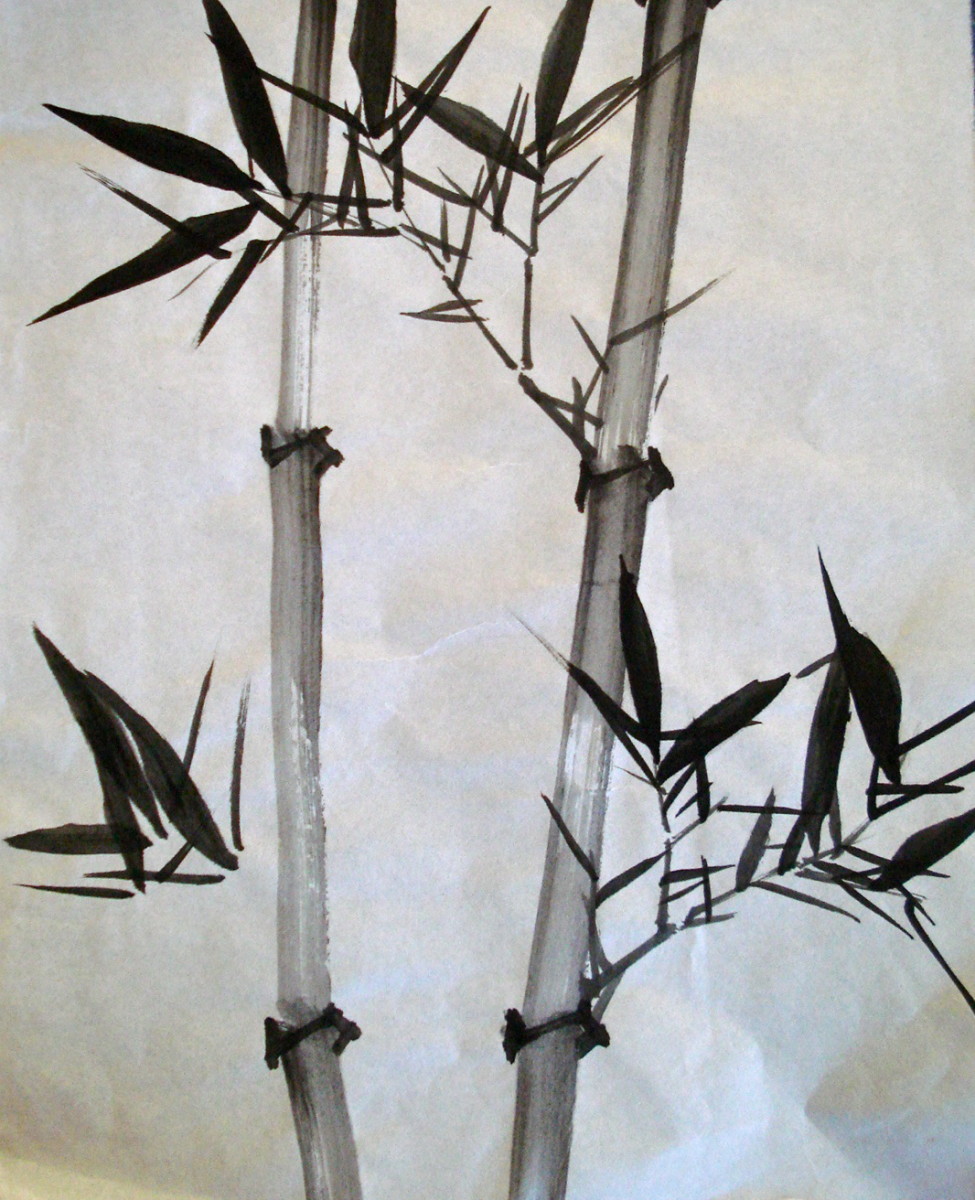This detailed black, gray, and white close-up image showcases a Chinese watercolor painting of bamboo stalks, exuding an ethereal quality. Two prominent, narrowly segmented bamboo stalks dominate the composition, each section meticulously rendered in charcoal gray with darker, black rings. The leaves, predominantly dark to almost black, extend elegantly from each segment, some appearing unattached and suspended in mid-air, adding a surreal element to the artwork. The background suggests a cloudy ambiance, enhancing the mystical atmosphere. With approximately fifteen distinct leaves of varying sizes, the composition reflects both intricate detail and artistic abstraction, capturing the essence of traditional Chinese brush painting.